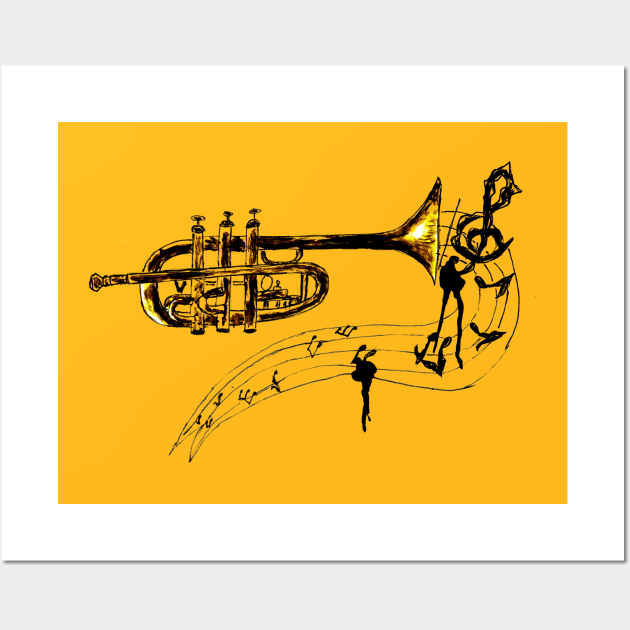This detailed artwork features a hand-drawn trumpet, elegantly displayed within a vibrant yellowish-orange rectangle bordered by a thick white frame. The trumpet's mouthpiece faces left, while its bell, the larger opening, points right. This intricately sketched instrument, marked by curves that twist twice and crowned by three valves, sits against a light gray backdrop encompassing the entire image. From the bell of the trumpet, a cascade of black musical lines swirls outward, weaving through and around, symbolizing the flow of music from larger to smaller notes. These lines not only carry music notes but also intertwine with the black pencil outlines of two different people, creating a harmonious interplay of music and human figures. The overall effect is a vivid, dynamic representation, merging musical and visual art in a meticulously sketched composition.